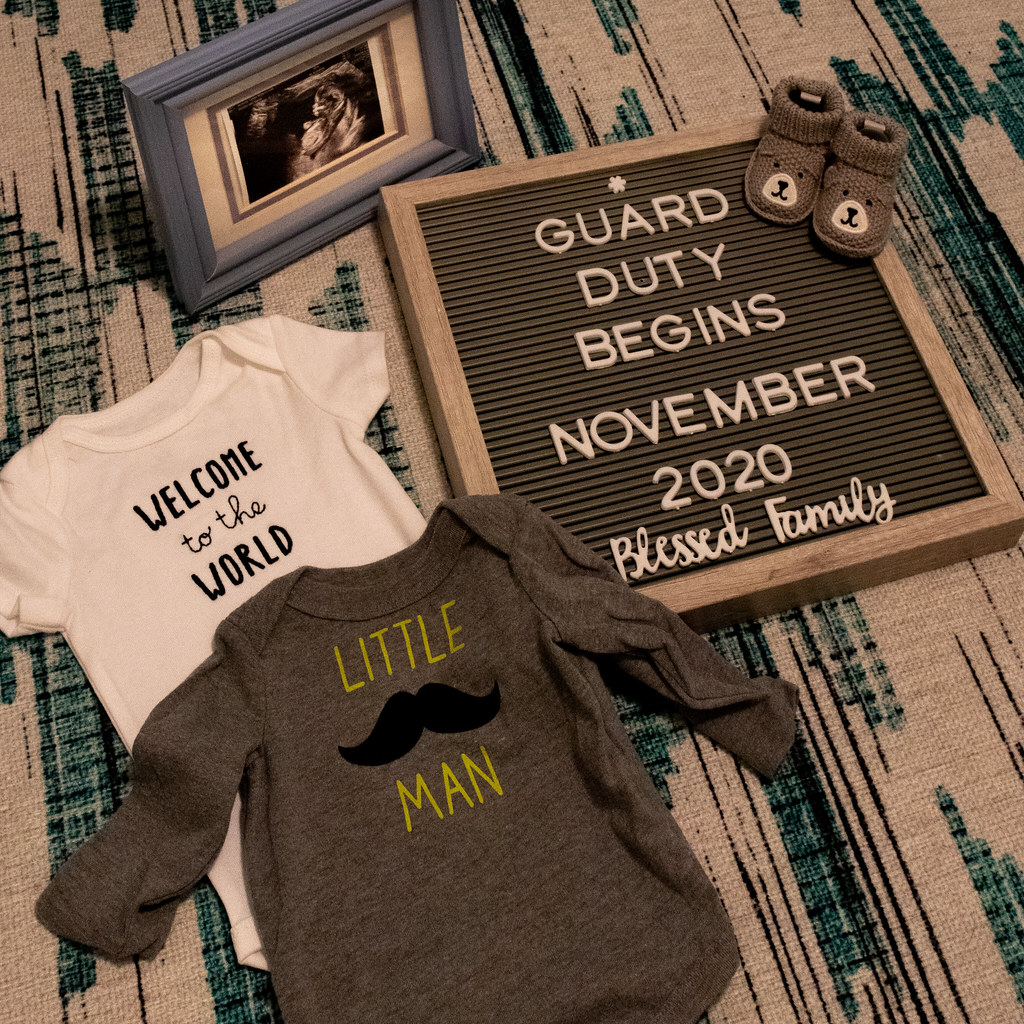The baby announcement photo is set against an ornate burlap fabric with dark green and black stripes. In the top left corner, a light blue framed picture showcases an ultrasound image. Below this, a white onesie with "Welcome to the World" written in black letters lies on the fabric. A gray long sleeve onesie with "Little Man" written in green letters and a mustache illustration rests on top of it. To the right, there is a word board with a light wood frame that reads "Guard Duty Begins November 2020" in clear letters, and "Blessed Family" in cursive. In the upper right corner of this board, a pair of light brown baby booties with bear faces adds a charming touch to the scene, emphasizing the joyful news of an upcoming addition to the family.